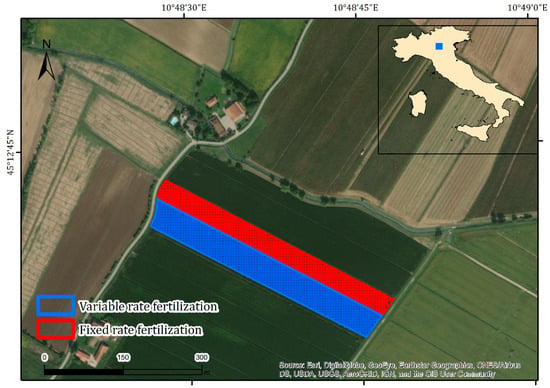This is a digitally enhanced, full-color aerial photograph taken outdoors during the day, showcasing an experimental maize production site at the Experimental Farm of the Department of Agriculture, Environmental Sciences, University of Milan, Italy. The image, in a square format with a very thin black border, captures varying fields of different textures and colors.

A small, inset map in the upper right corner highlights the location within Italy, depicting the country in brown against a light background. The focal point of the photograph is divided into two distinct areas: a blue box labeled "variable rate" and a red box labeled "fixed rate," each representing different fertilization methods—variable and fixed rates of nitrogen top-dressing, respectively.

The blue section demonstrates a fertilization method that adjusts the nitrogen levels based on specific needs, while the red section shows a uniform application of nitrogen. Overlaid text on the image, which includes numerical data and possible geographical coordinates, further delineates the areas and their specific treatments. The experimental setup aims to illustrate that varying nitrogen application rates did not negatively impact maize yields, providing valuable insights into sustainable agricultural practices.